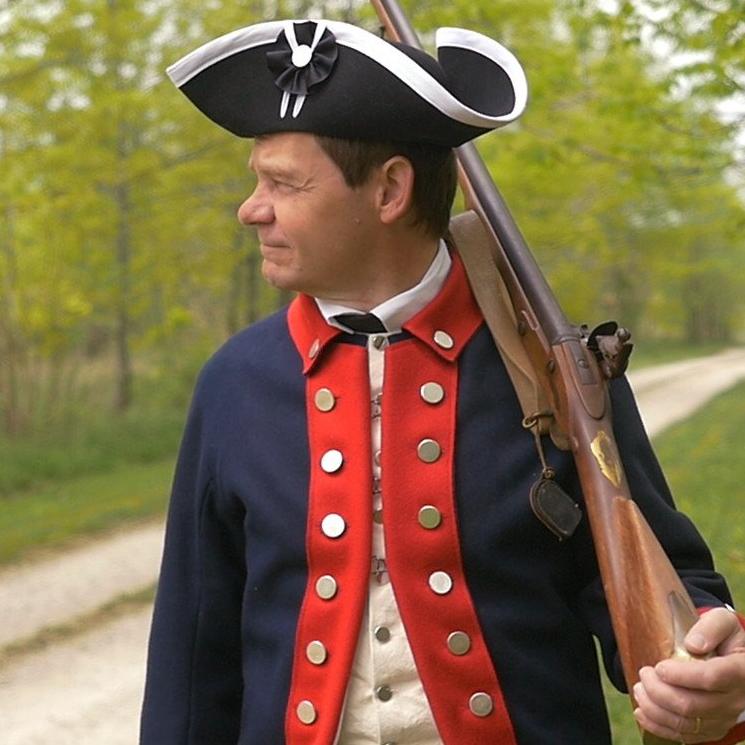The image features a close-up, vertically oriented shot of a man dressed in a historically inspired Minuteman or Revolutionary War reenactment outfit. He dons a dark blue coat with distinctive red trim and gold buttons running down the front. Underneath, he wears a white vest with silver buttons, a white shirt, and possibly a tie. A striking black tricornered hat with a white border and a black-and-white ribbon adorns his head, evoking a Paul Revere-like appearance. The man cradles an old-style musket over his shoulder, complete with a brown strap and a medallion near its base. He is positioned on a grassy expanse beside a dirt road, with a lush, forested area featuring abundant green leaves in the background. The man's right hand is visible resting on the butt of his rifle.